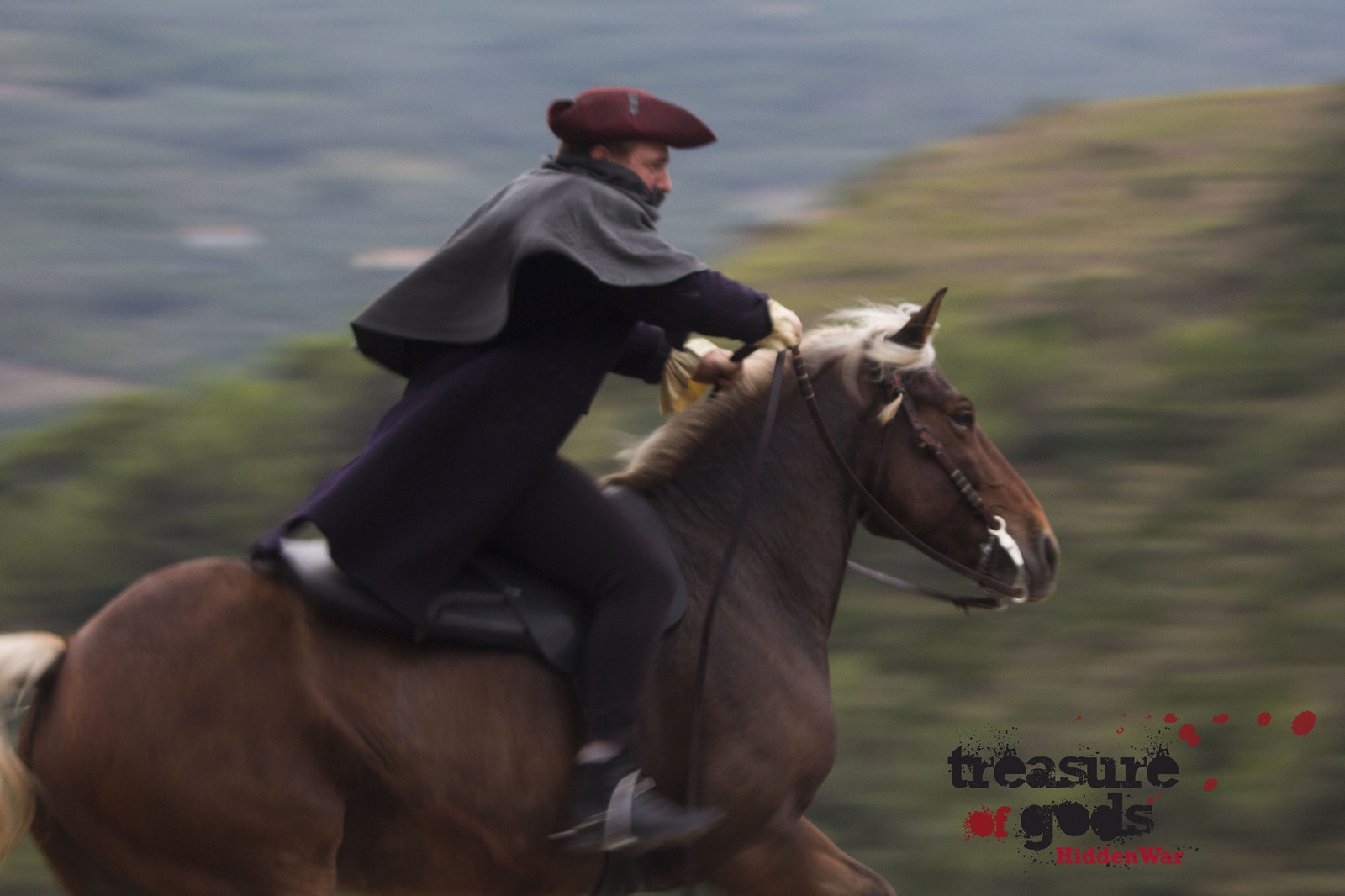The image depicts a person reminiscent of Paul Revere, riding a large, brown horse with a striking blondish-white mane and tail at full gallop. The rider is donned in attire evocative of the 16th or 17th century, with a notable reddish-colored tricorn hat that shades his face. He wears a light gray cape draped over his shoulders, a long-sleeved brown jacket that flutters with the speed, dark brown or black pants, and dark boots with a glimpse of the ankle visible. His feet are securely in the stirrups as he grips the reins tightly, leading the horse through what appears to be a hilly countryside. The background is a blur of green grass, brown dirt, shrubbery, and scant short trees, indicating the rapid motion and outdoor setting of the shot. In the bottom right corner, the text "Treasure of the Gods" is prominently displayed in black letters with "Hidden War" written in small red letters below, suggesting a possible title for a show or film.